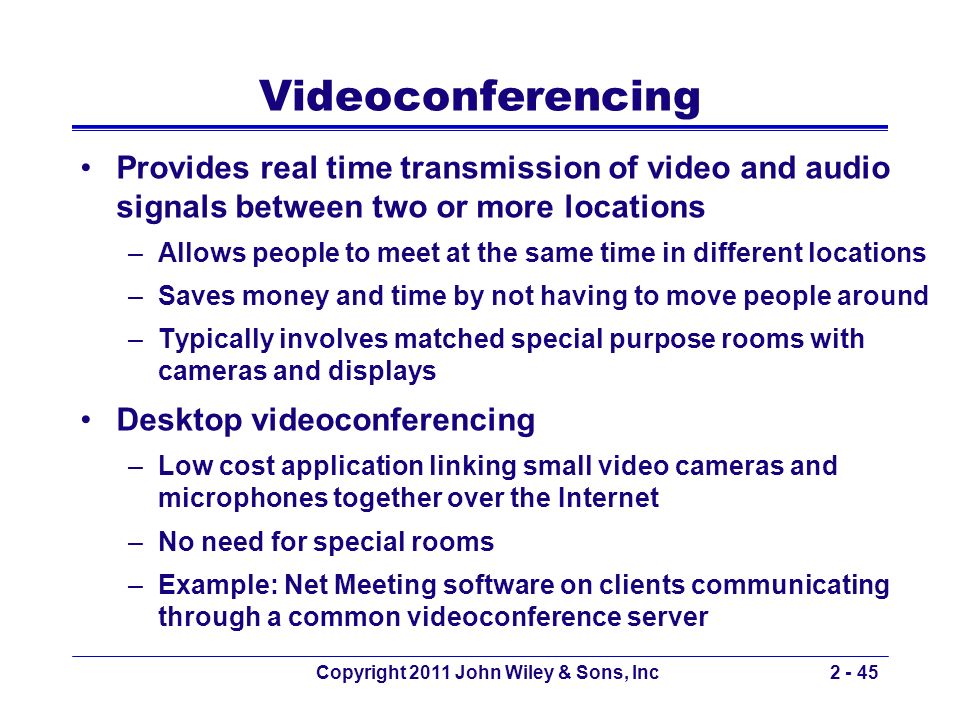This image depicts a PowerPoint or Google Slides presentation slide with a white background, featuring only blue text and no images. The slide is titled "Videoconferencing" and is separated by a horizontal blue line. The first primary bullet point reads "Provides real-time transmission of video and audio signals between two or more locations," and it elaborates with sub-points that highlight its benefits: allowing people to meet simultaneously in different locations, saving time and money by avoiding physical travel, and typically utilizing specially equipped rooms with cameras and displays. The second main bullet point is titled "Desktop Videoconferencing," describing it as a low-cost solution that links small video cameras and microphones over the Internet, negating the need for special rooms. It provides an example of net meeting software allowing clients to communicate via a common videoconference server. The slide ends with a horizontal blue line and a small text note at the bottom right, stating "Copyright 2011, John Wiley & Sons, Inc.," followed by "2-45."